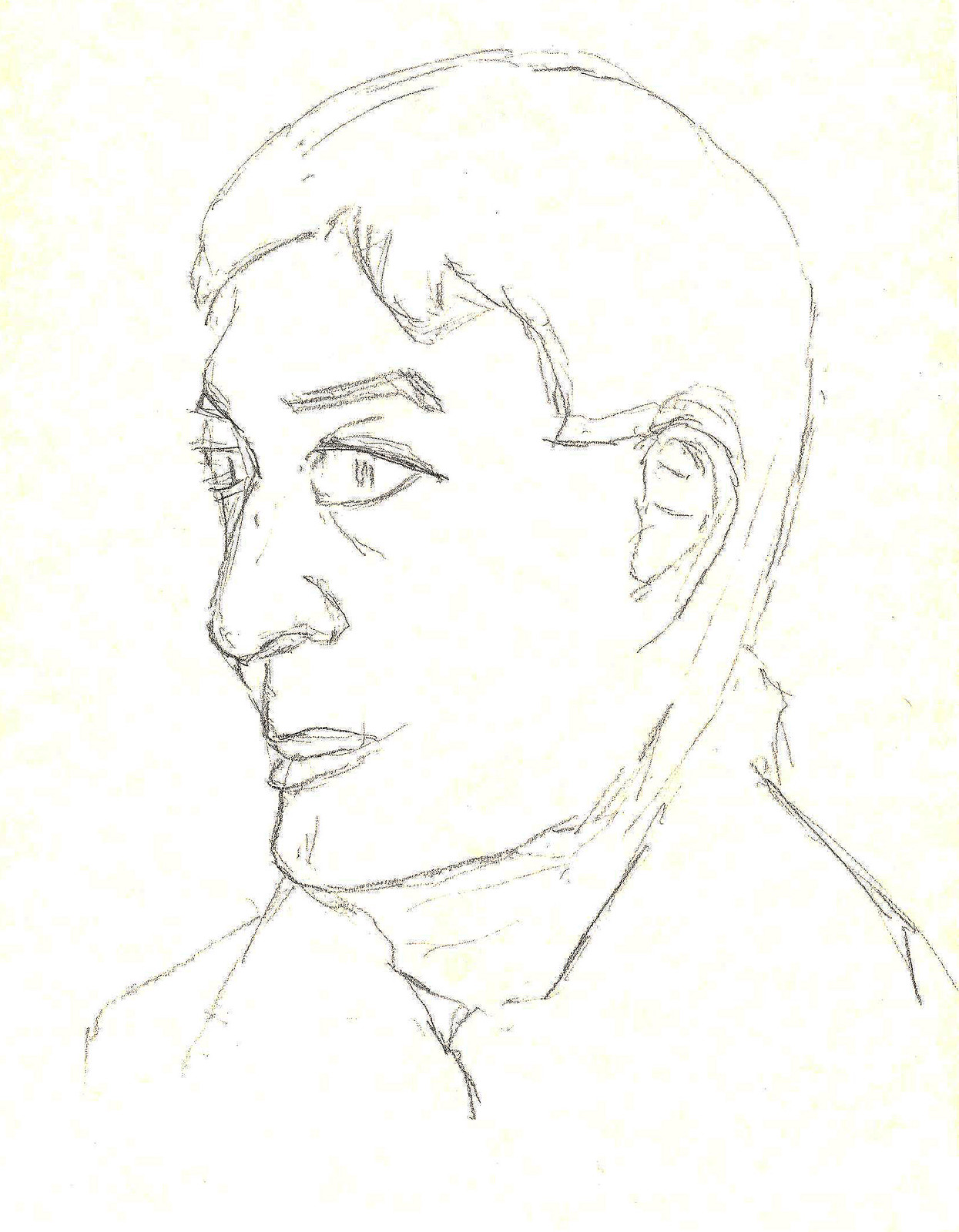A monochromatic drawing of a person in black ink is presented against a background of white with yellowish tones. The artwork captures the left profile of the individual's face and left shoulder. Distinct facial features, including the left ear, eyes, nose, lips, and a closed mouth, are clearly depicted. The hair is intricately drawn, and the neckline gently transitions into a partial view of the shoulders. The drawing stops just above the chest, leaving the lower part of the body unseen. The minimalistic yet detailed rendering highlights the contemplative expression of the subject, standing out starkly against the light background.